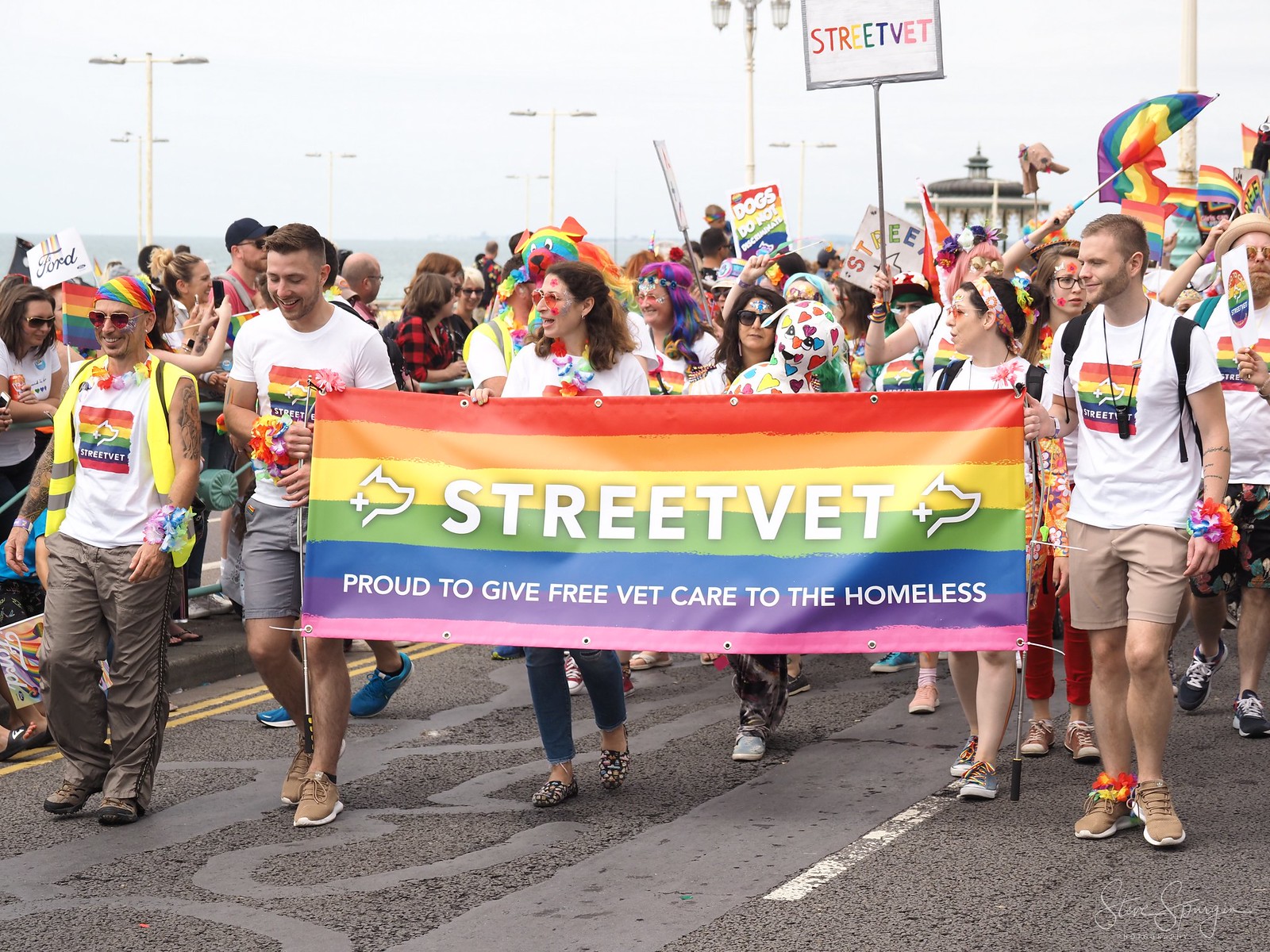In this image, a large group of people is marching down an asphalt street, which you'd typically see cars driving on. The people are centered in the middle of the image, holding a giant rainbow flag with the text "Street Vet, proud to give free vet care to the homeless" written in white. The crowd, many of whom are wearing rainbow-colored clothing, Street Vet branded white shirts with a rainbow logo and a dog outline, are either waving rainbow-colored signs or flags. They appear to be participating in a parade, likely a Gay Pride festival, given the prominent rainbow symbols. The setting is outdoors, in the middle of the day. In the background, the top of the image shows a body of water, a distant sky, and several streetlights, suggesting a beachy environment. The colors visible include red, orange, yellow, green, blue, purple, pink, white, black, and gray.